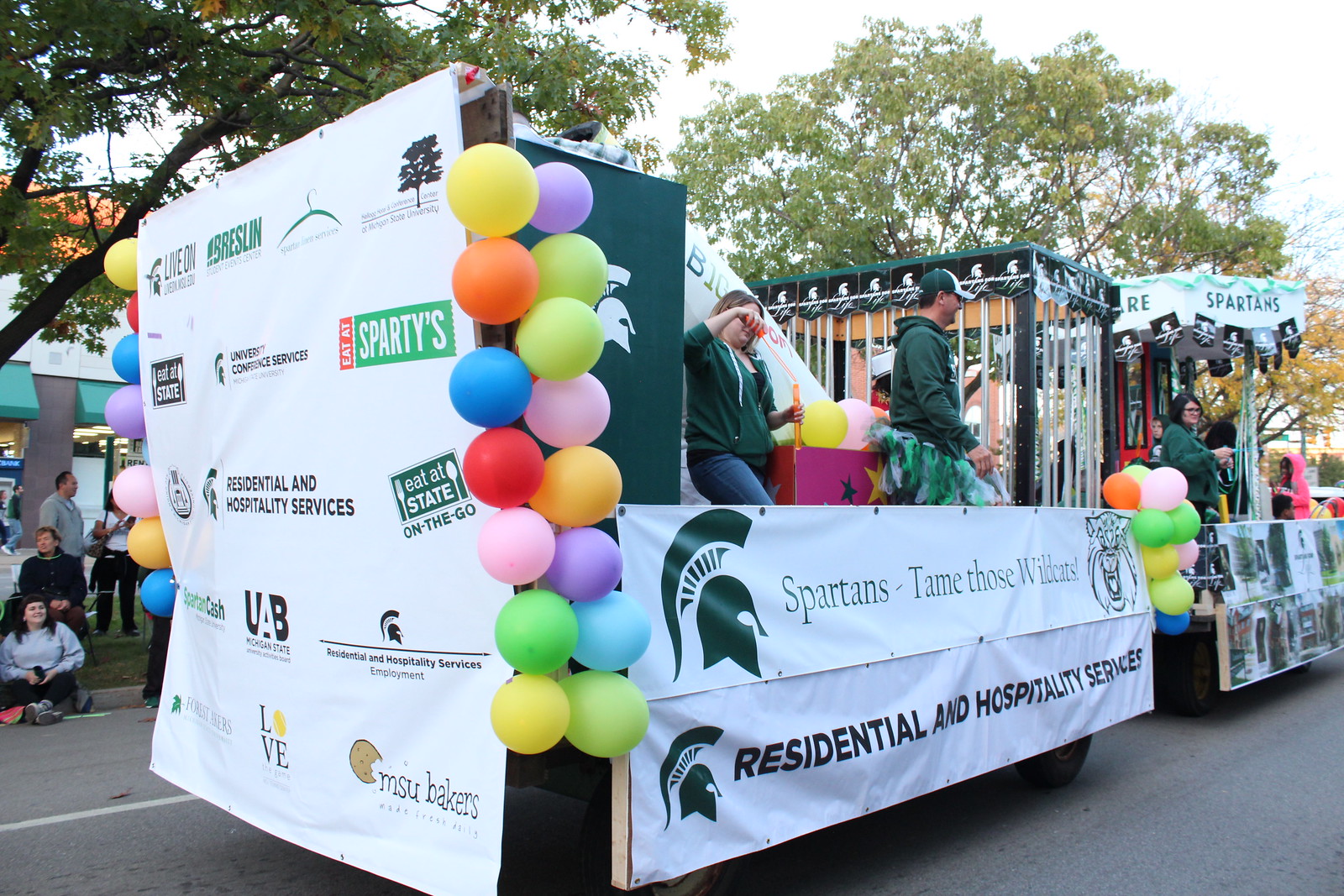This outdoor photograph captures a vibrant parade scene on a sunlit city street, filled with details and movement. Central to the image is a large, rectangular float, viewed at a three-quarter angle as it progresses from left to right. This open-air, truck-chassis float is predominantly decorated in green and white, representing the Michigan State Spartans.

The float's right rear corner is festooned with colorful balloons arranged in two vertical columns, featuring a spectrum of colors including yellow, purple, orange, green, blue, pink, red, and more. There's a similar balloon arrangement at the front right corner of the float. Along the side, two banners display the Spartan helmet icon and messages. The top banner has text that reads "Spartans Tame Those Wildcats," accompanied by another logo. The lower banner, which covers the wheels, bears the phrase "Residential and Hospitality Services" in black lettering on a white background.

On the float, a man and a woman, both wearing green hoodies and jeans, stand out. The man, positioned at the forward right corner, also sports a green and white baseball cap and has dark brown hair. The woman, whose face is obscured, has her hand raised. At the center of the float is a pink table.

To the left edge of the image, spectators line the street, with some sitting on the curb and others standing on the sidewalk, attentively watching the parade. Behind them, buildings and trees line the street. The background reveals a canopy of trees above the floats, indicating a sunny but slightly washed-out sky. Another parade float is visible ahead in the distance, though too far to discern details. This lively scene captures the essence of a community coming together to celebrate amidst a backdrop of festivities and camaraderie.